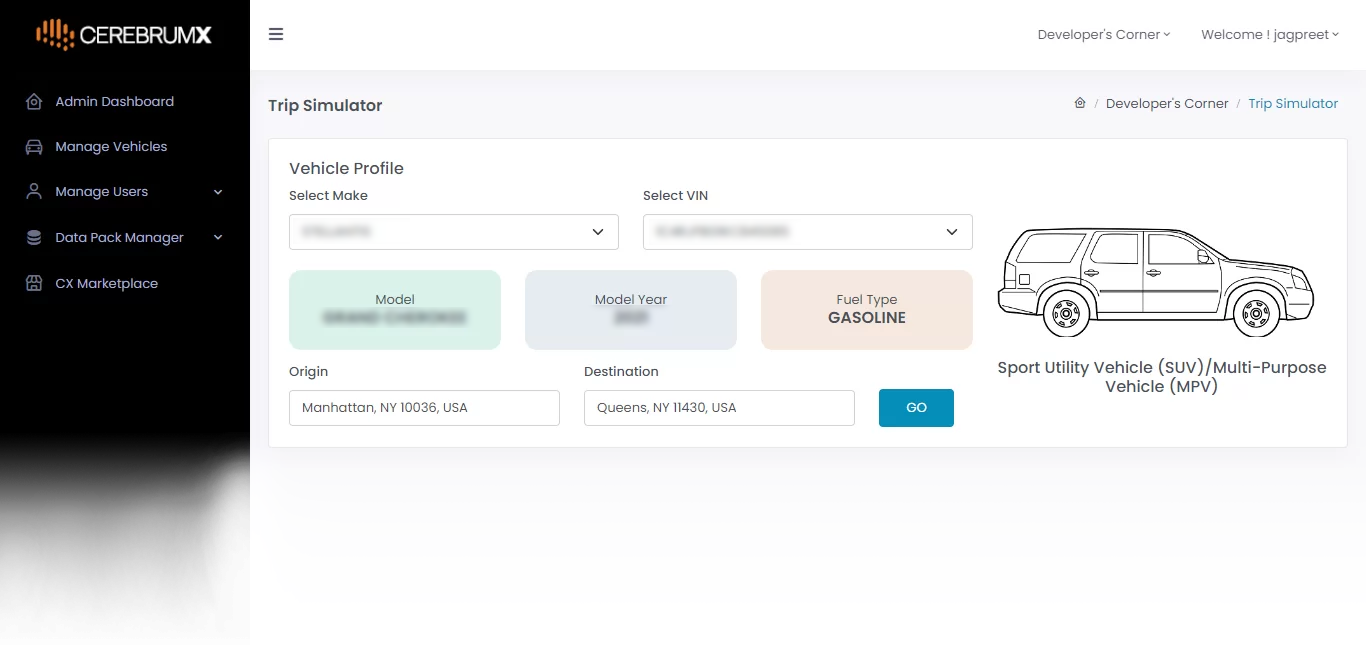This is a screenshot from the Cerebrum X trip simulator interface. On the left side, occupying approximately 10-15% of the image, there is a vertical black banner that transitions into white as it moves downward. The top of this banner displays the "Cerebrum X" logo, with vertical orange dashes indicating different sections below it. These sections include "Admin Dashboard," "Manage Vehicles," "Manage Users," "Data Pack Manager," and "CX Marketplace," each with corresponding icons. Dropdown arrows appear next to the "Manage Users" and "Data Pack Manager" sections.

On the right side, against a white background, is a detailed interface. At the top left, there is a hamburger menu icon, and to the right, it says "Developers Corner" and "Welcome Jagpreet." Below this header, "Trip Simulator" and "Developers Corner Trip Simulator" are written in blue hyperlinked text.

Further down, there is a "Vehicle Profile" section with dropdown fields for selecting the vehicle's make, VIN, model, model year, and fuel type. The "Model" field is highlighted in green, the "Model Year" in gray, and the "Fuel Type" in taupe. Below these fields are the "Origin" and "Destination" settings filled with "Manhattan, New York" and "Queens, New York," respectively, followed by a "Go" button.

To the right of these settings, there are descriptions and an image of an SUV, labeled as "Sport Utility Vehicle (SUV)" and "Multi-Purpose Vehicle (MPV)."